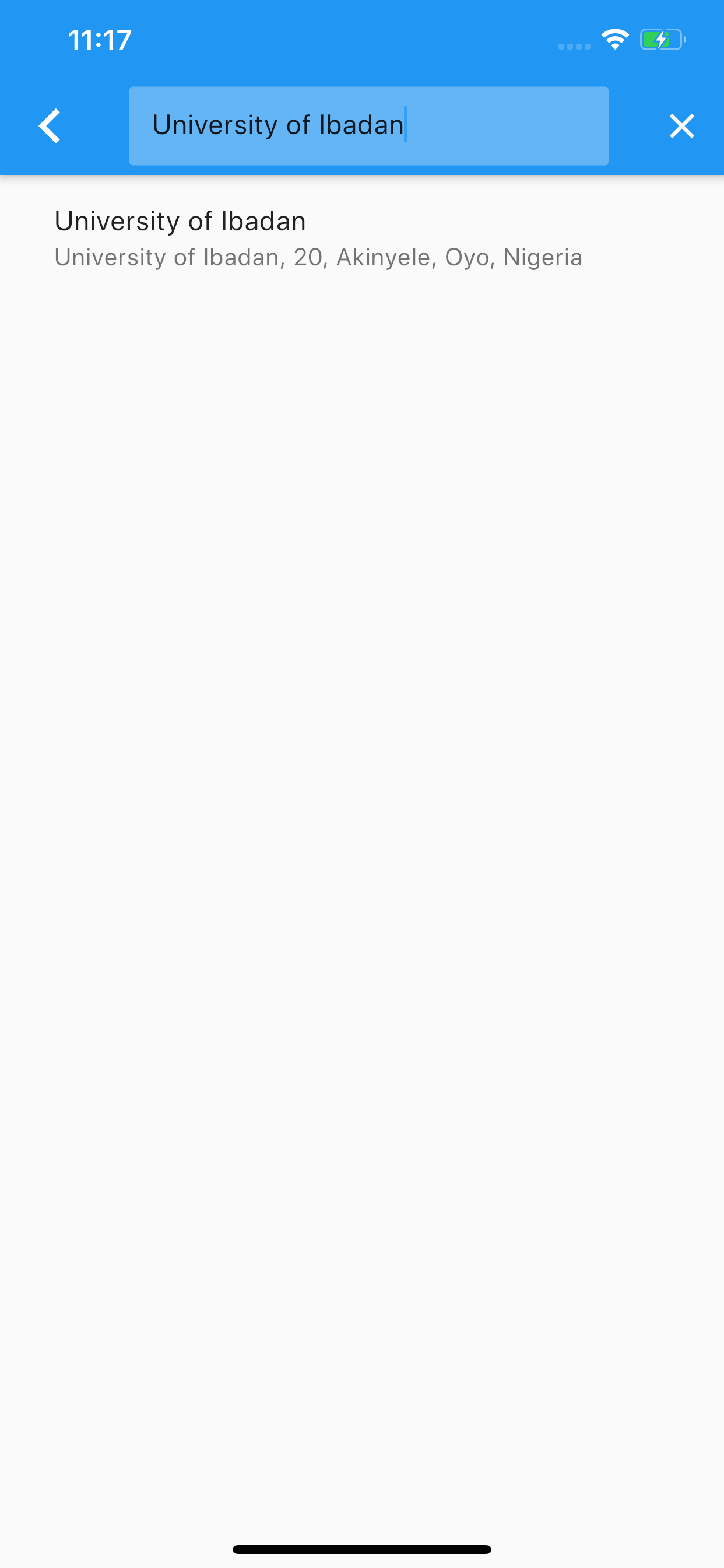The image features a medium blue bar at the top where the time is displayed as 11:17. Inside a slightly darker blue rectangle within the bar is the text "University of Ibadan" followed by a vertical separator line. In the top right corner, a battery icon indicates it is slightly less than half full, with a small white lightning bolt symbol inside. 

Below the blue bar is a white 'X' icon. The main portion of the image prominently features the text "University of Ibadan" repeated multiple times. In a lighter gray color beneath, it reads "University of Ibadan, 20, Akinyele, Oyo, Nigeria," with the 'O' in 'Oyo' capitalized. 

At the very bottom of the image, there is a short, approximately three-inch long black horizontal line. Just below this line, the text "University of Ibadan, 20, Akinyele, Oyo, Nigeria" appears again.